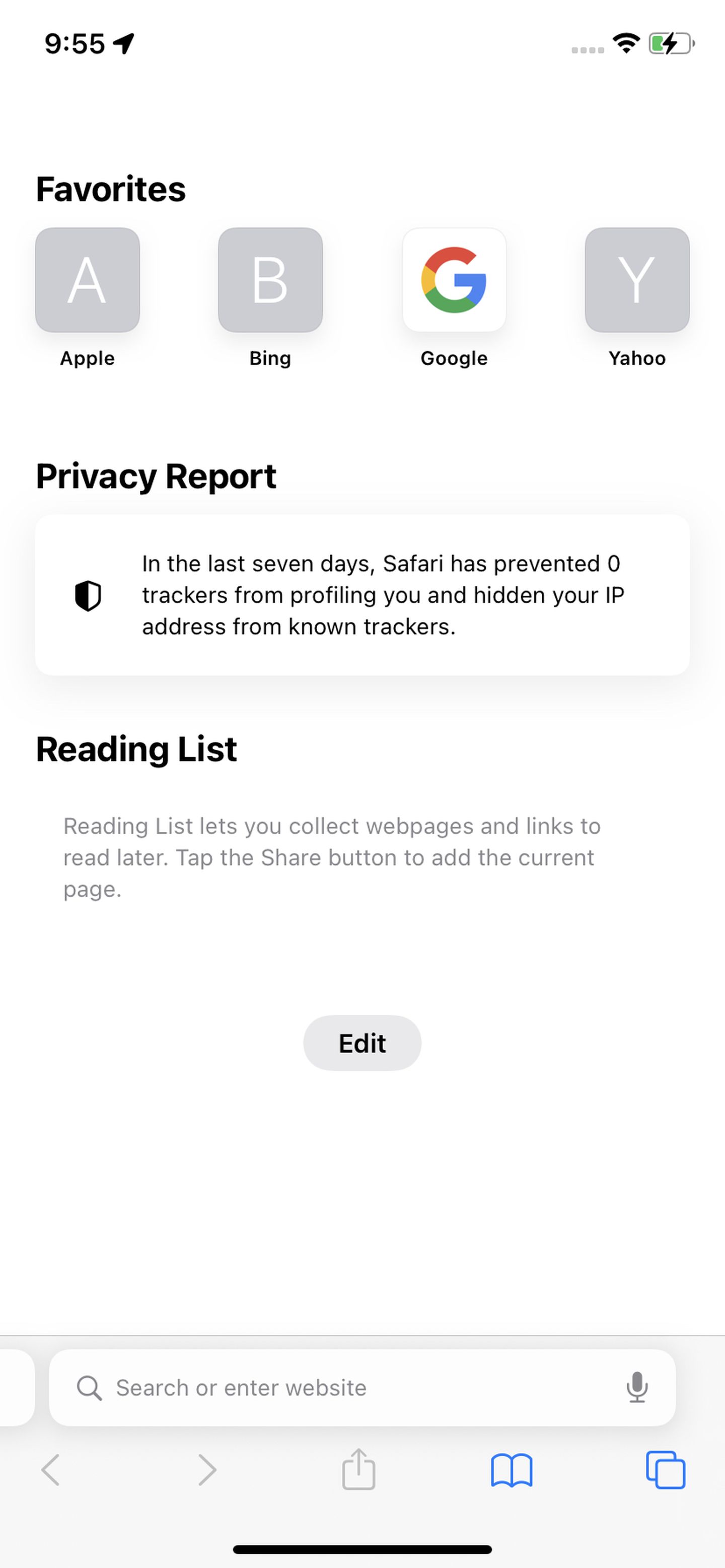Screenshot Description: 

The screenshot depicts a smartphone screen with a series of app icons and information panels. The time displayed is 9:55, and the battery icon shows that it is charging. 

At the top, there's a "Favorites" section featuring several app icons each inside a square: 
- Apple, represented by an 'A' in a square.
- Bing, represented by a 'B' in a square.
- Google, represented by a stylized 'G' in a square with its signature colors (blue, red, yellow, and green).
- Yahoo, represented by a 'Y' in a square.

Below these icons, there is a "Privacy Report" section indicating that Safari has prevented zero trackers from profiling the user and has hidden the user's IP address from known trackers over the last seven days.

Next, a "Reading List" section explains its function: it helps users collect web pages and links to read later. Users can add the current page to the reading list by tapping the share button. An "Edit" button within a gray oval is shown in black text.

At the bottom, there's a search bar with a magnifying glass icon on the left and a microphone icon on the right. Further down, there is a navigation bar with a left arrow, a right arrow, a share button, a book icon, and an icon depicting two overlapping squares.